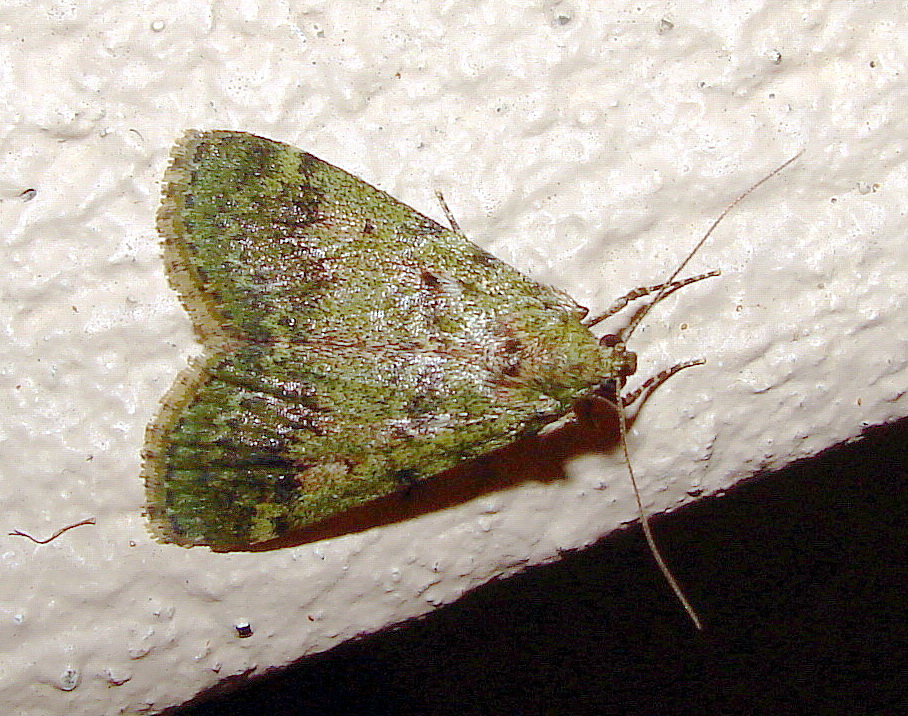The image features a green moth perched on a jagged, white-painted concrete surface that seems to be part of an outdoor building. The moth, displaying various shades of green in a near-camouflaged pattern, has two large closed wings and long antennae extending from its head. Its body is oriented with the head to the right and wings to the left. You can see three legs in total: two front legs protruding forward near its face and one rear leg visible underneath a wing. The bottom right corner of the photo contrasts sharply with the rest of the image, being dark black and highlighting the structure's irregular texture.